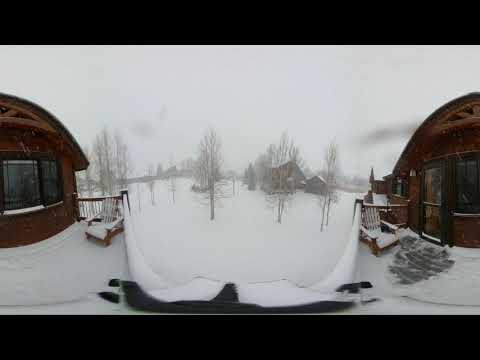The image, framed by a black header and footer, captures a snowy outdoor scene during the daytime, featuring two nearly identical wooden buildings with rounded roofs and log cabin-like structures. Both buildings, dark brown in color, are situated on the left and right sides of the image. The building on the left has two large windows with black frames and a snow-covered deck, on which sits a dinner chair blanketed in snow. A wooden railing extends and curves around the deck area. The building on the right features a single door made of two panes of glass and also has a snow-covered deck with a chair, where a small patch of snow has been brushed aside, revealing the ground beneath. In the middle ground, the snow continues to cover the entire area, while a line of barren trees stretches across the background. Further into the distance on the right side, a house with an arched roof stands next to a smaller structure with a similar arched design. The sky is completely gray, creating a somber and wintry atmosphere, with a single darker gray spot above the house on the right.